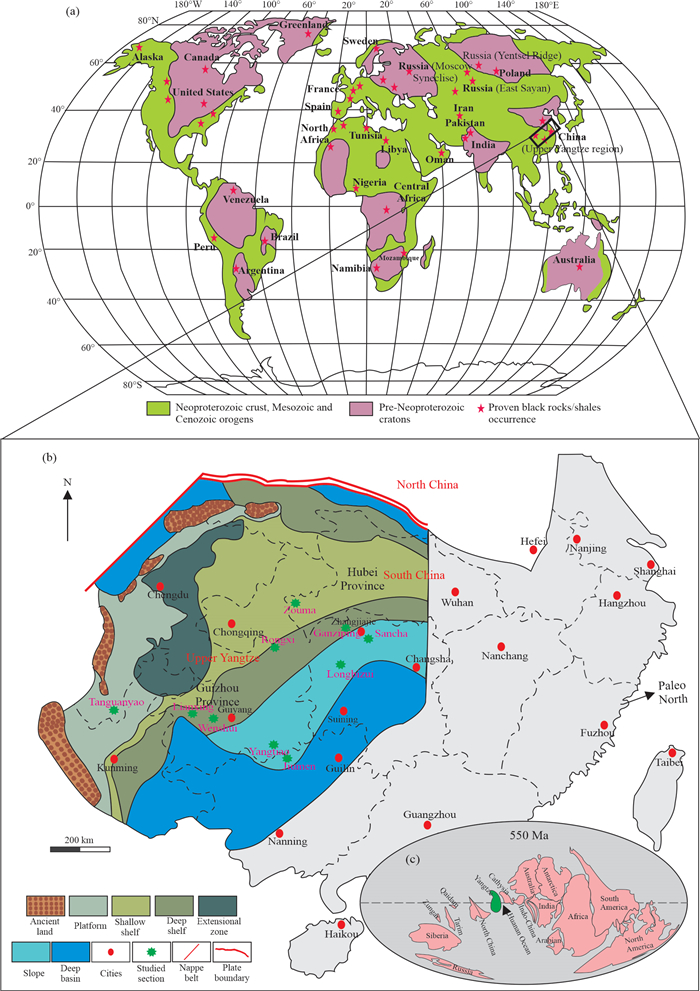The image presents two maps: an upper depiction of the entire world in an unknown projection showing continents and countries, with North and South America on the left, Africa, Europe, and Asia in the center, and Australia at the bottom right. Distinctive features include curved latitude and longitude lines. Two lines point from the main map to a detailed zoomed-in map below, focusing on North China. This lower map highlights various provinces and cities, including Guangzhou, Wuhan, and Taiwan, with tiny and almost unreadable text.

The zoomed-in section of North China is intricately color-coded and includes a key. The regions are shaded in colors to represent geologic periods and structures: purple for pre-Neo-Proterozoic cratons, green for Neo-Proterozoic to Cenozoic formations, brown for ancient land, greenish-gray for platforms, shades of blue for shallow to deep basins, and dark to light greens for different shelves and zones. Red stars mark proven black rocks/shales occurrences, and green stars indicate studied sections. Additionally, the map shows important geological features like nappes and plate boundaries, marked with red lines at the top of North China.